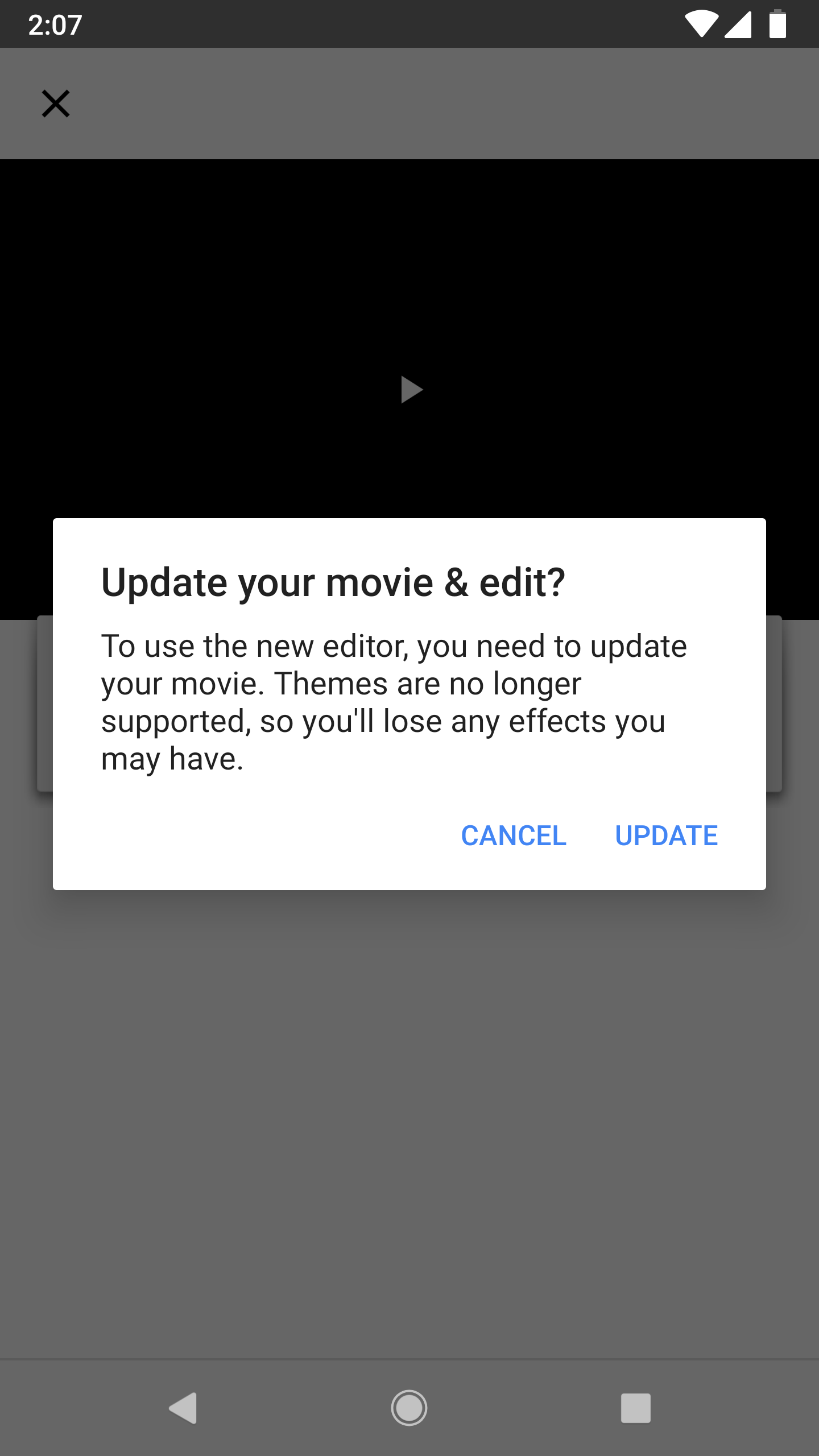Screenshot of a smartphone displaying an update notification for a movie editing app, set against a light-themed interface. The top section of the screen shows the status bar with full Wi-Fi signal, full battery, and other icons, including “207” indicating the time. The central part of the screen features a black rectangle with a play button, symbolizing a video’s thumbnail. Below it, a notification box in white reads: "Update your movie and edit. To use the new editor, you need to update your movie. Themes are no longer supported, so you'll lose any effects you have. Cancel. Update." The bottom-most section of the screen is also white, contributing to the overall light theme of the interface.